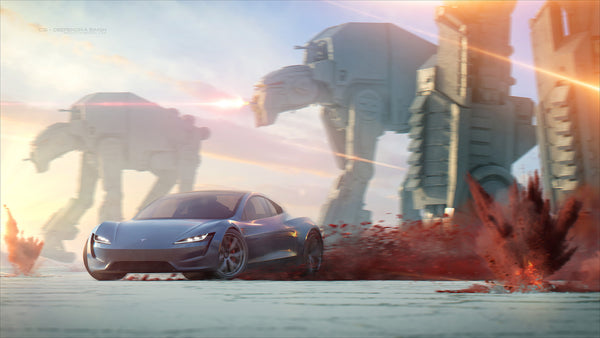The image appears to be a computer-generated or heavily edited artwork depicting an intense scene reminiscent of a Star Wars battle. Dominating the foreground is a sleek blue sports car skidding across a white surface, possibly snow, and kicking up clouds of red dust or dirt. The car's dynamic movement suggests it's driving hastily toward the left side of the image, adding to the sense of urgency and action. The car features distinctive headlights resembling slashes or eyes with dark windows, giving it a futuristic and aggressive appearance.

In the background, two colossal AT-AT walkers from the Star Wars universe are prominently visible, firing red laser beams into the sky and possibly engaging in combat. Additionally, the legs of another AT-AT can be seen in the foreground, intensifying the chaotic atmosphere. An explosion is also noticeable in one corner, contributing further to the red dust clouds and adding to the visual drama. The sky is light blue with scattered clouds, enhancing the contrast between the serene backdrop and the violent battle scene below. Although partially obscured, there appears to be illegible text at the top left corner of the image. Overall, the scene is a vivid and detailed portrayal of a futuristic car navigating a perilous Star Wars-like battleground.